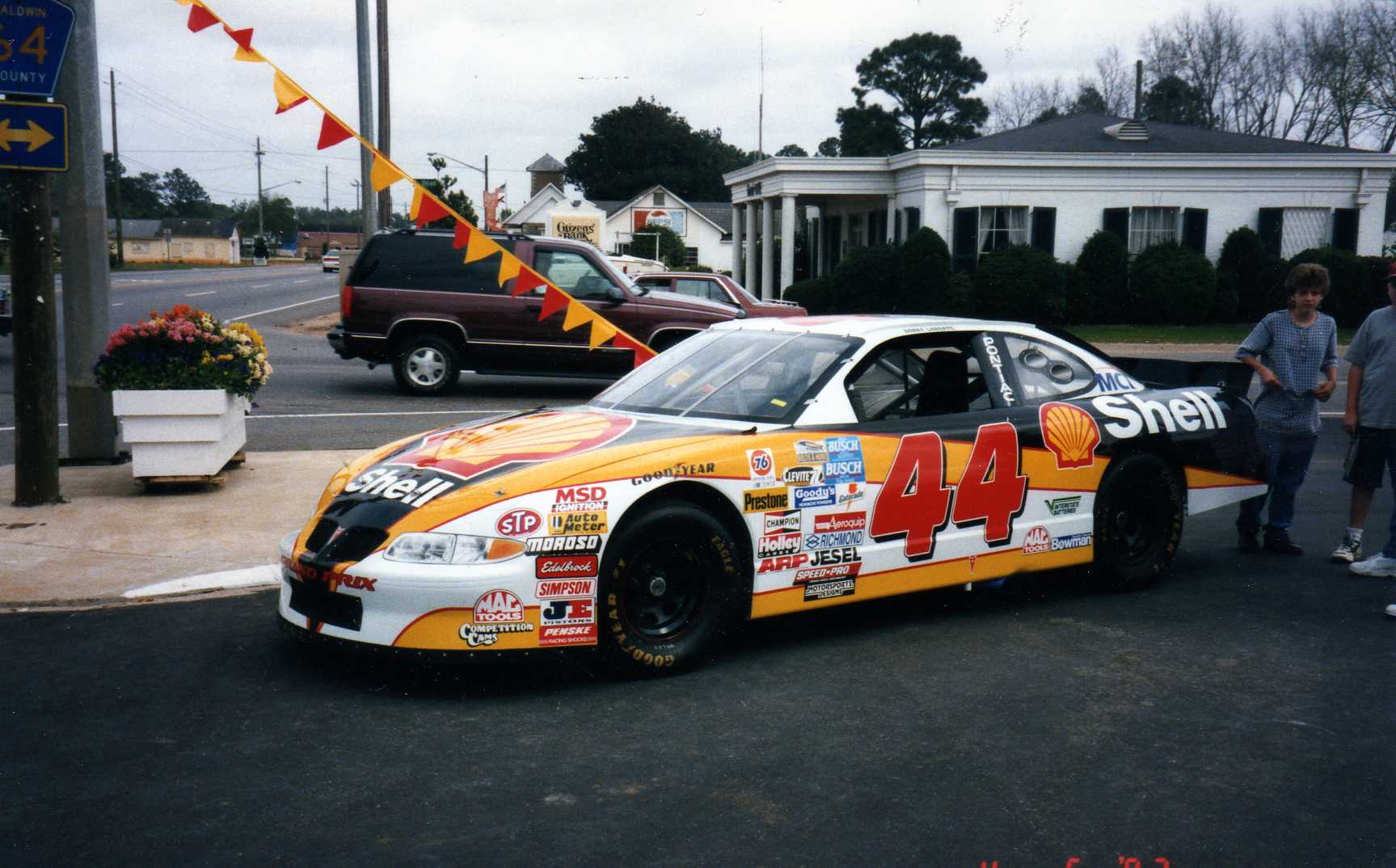The photograph features a race car that resembles a NASCAR vehicle, parked on a dark asphalt surface beside a cement sidewalk. The car is predominantly white, yellow, and black, prominently displaying the Shell logo in red and yellow on the hood and rear quarter panel, with bold white text reading "Shell" below the emblem. The number 44, in bright red, is visible on the driver’s door, surrounded by various decals and sponsor logos including 76, Prestone, Busch, STP, MacTools, Simpson, JE, Jessel, ARP, Holley, and others.

To the right of the car, partially cropped out of the frame, are two people. The man wears a light blue shirt and blue jean shorts, though only half of him is visible. Next to him is a woman in a blue and white button-up shirt with sleeves rolled up and blue jeans. Surrounding the car, the black tires bear gold "Goodyear" lettering.

In the background, a single-story white building, resembling a bank, features windows with curtains, a small portico supported by four columns, and manicured bushes. Behind this building, a row of passenger vehicles includes a maroon SUV and a maroon four-door car. Further back, a retail area with signs such as "Pepsi" and potentially "Genesis Taxes" is visible.

A couple of trees and a few telephone poles line the right side of the image, while on the left, a four-lane street and a distant house are observable. The sky is overcast, creating a muted gray backdrop for the scene. Framing the car on the cement sidewalk, a white flower box holds vibrant yellow and orange flowers, and overhead, yellow and red banners stretch from the car towards the building’s roof.